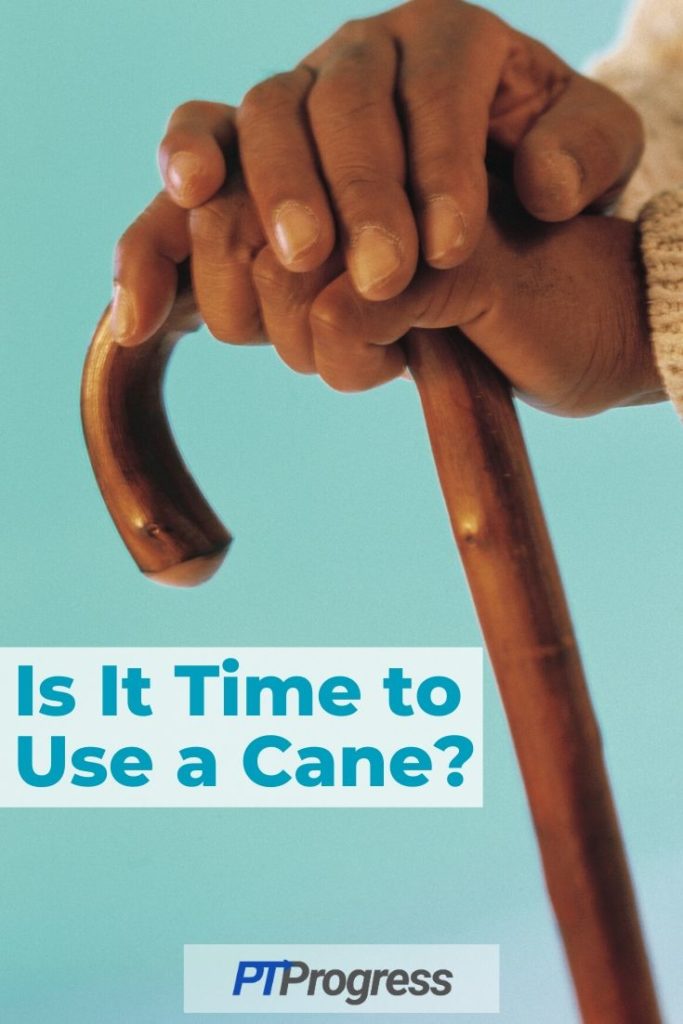This advertisement for PT Progress features an evocative image set against a mint or seafoam green background. Dominating the top right of the image, a pair of hands rests gently on a medium brown wooden cane, the hands suggestively belonging to an elderly individual, possibly female, clad in a tan sweater. The positioning of the hands and cane create a diagonal line leading from the center towards the bottom right of the photo, emphasizing stability and support.

On the left-hand side near the bottom, a white box with bold blue lettering poses the thought-provoking question: "Is it time to use a cane?" Below this, another white box centers the tagline for PT Progress with "PT" in large blue letters and "progress" in gray, indicating the organization behind the ad. The overall palette features harmonious shades of blue, brown, tan, white, gray, and turquoise, coming together to create a comforting and reassuring visual cue, reinforcing the message of seeking assistance when needed.